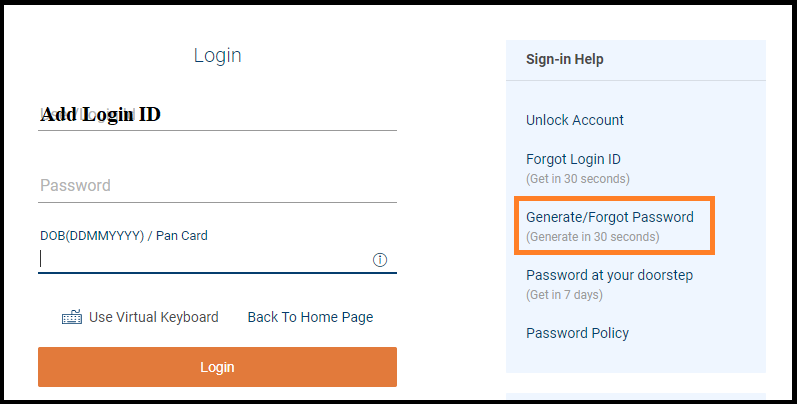The image is a partial screenshot of a webpage. The background is white, enclosed within a black rectangular outline, with dimensions wider than taller. 

On the left side, in very light gray font, the text "Login" is displayed. Below this, separated by a gray line, the bold black text "Add Login ID" is prominently shown. Underneath this, a space is reserved for user input, followed by another light gray line. Below this line, the light gray text "Password" appears, indicating where to input the password. Further down, yet another line separates this section from the "DOB" field, which stands for Date of Birth. In parentheses, "DDMMYYYY" specifies the desired format for the date of birth entry. 

At the very bottom of this section, an oblong, burnt orange button labeled "Login" in white font serves as the submission mechanism.

On the right side of the image, there is a light blue box. At the top, the text "Sign In Help" is displayed. Below this, in blue font, the options "Unlock Account" and "Forgot Login ID" are listed, with a parenthetical note in gray font stating "Get in 30 seconds". Further down, "Generate/Forgot Password" is shown in medium blue font, accompanied by "Generate in 30 seconds". This section is enclosed in an orange rectangular outline. Below this, in blue font, the text "Password at your door" appears, with a note indicating "Get in 7 days". Finally, at the very bottom of the box, "Password Policy" is listed.